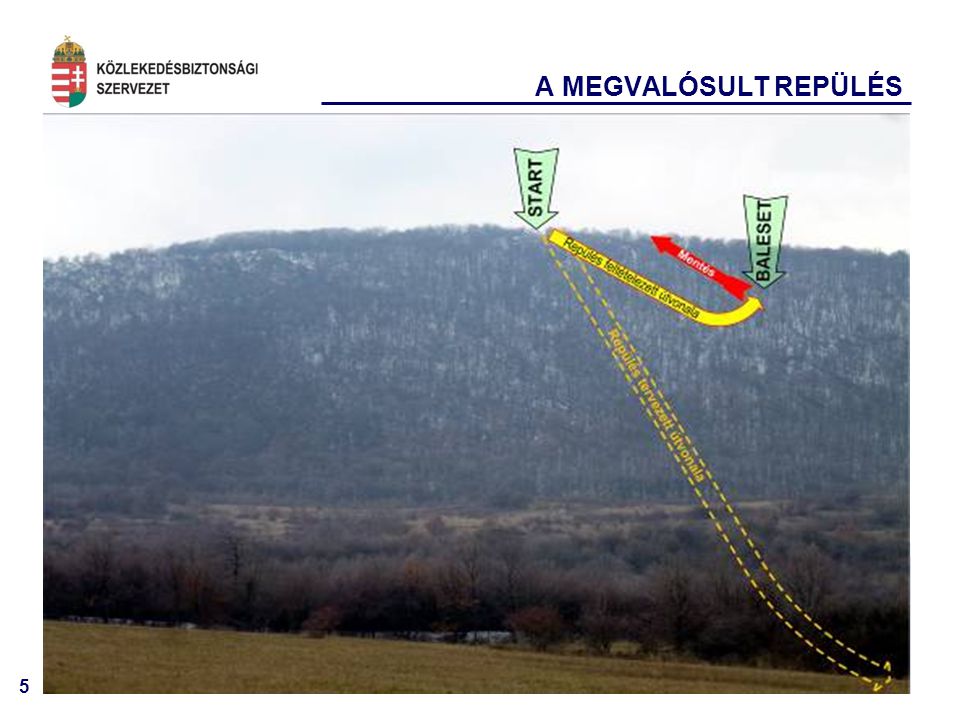The photograph showcases a scenic landscape with a mountainous background covered in trees, transitioning to a slightly lower hill adorned with more trees, and culminating in an open, grassy meadow in the foreground. The meadow appears to be in fall or winter, with brown, leafless trees dotting the area. Overlaid on this image is a complex diagram involving multiple arrows and text. 

At the top of the prominent mountain or hill, a green arrow labeled "start" points downward. A dashed yellow line extends from this starting point, with additional yellow arrows on a yellow background pointing right. A second green arrow labeled "ballast" directs attention downward towards these yellow elements. A red arrow curves upwards and leftwards from the ballast point, while another green arrow descends, interacting with the yellow pathway. 

Writing is present at the top of the image in a foreign language, possibly Scandinavian or Dutch. A distinctive emblem occupies the upper left corner, featuring horizontally striped red and white sections on the left and a white cross with two lines through it on the right. The diagram’s purpose remains unclear but suggests a directional or instructional theme possibly related to the landscape.